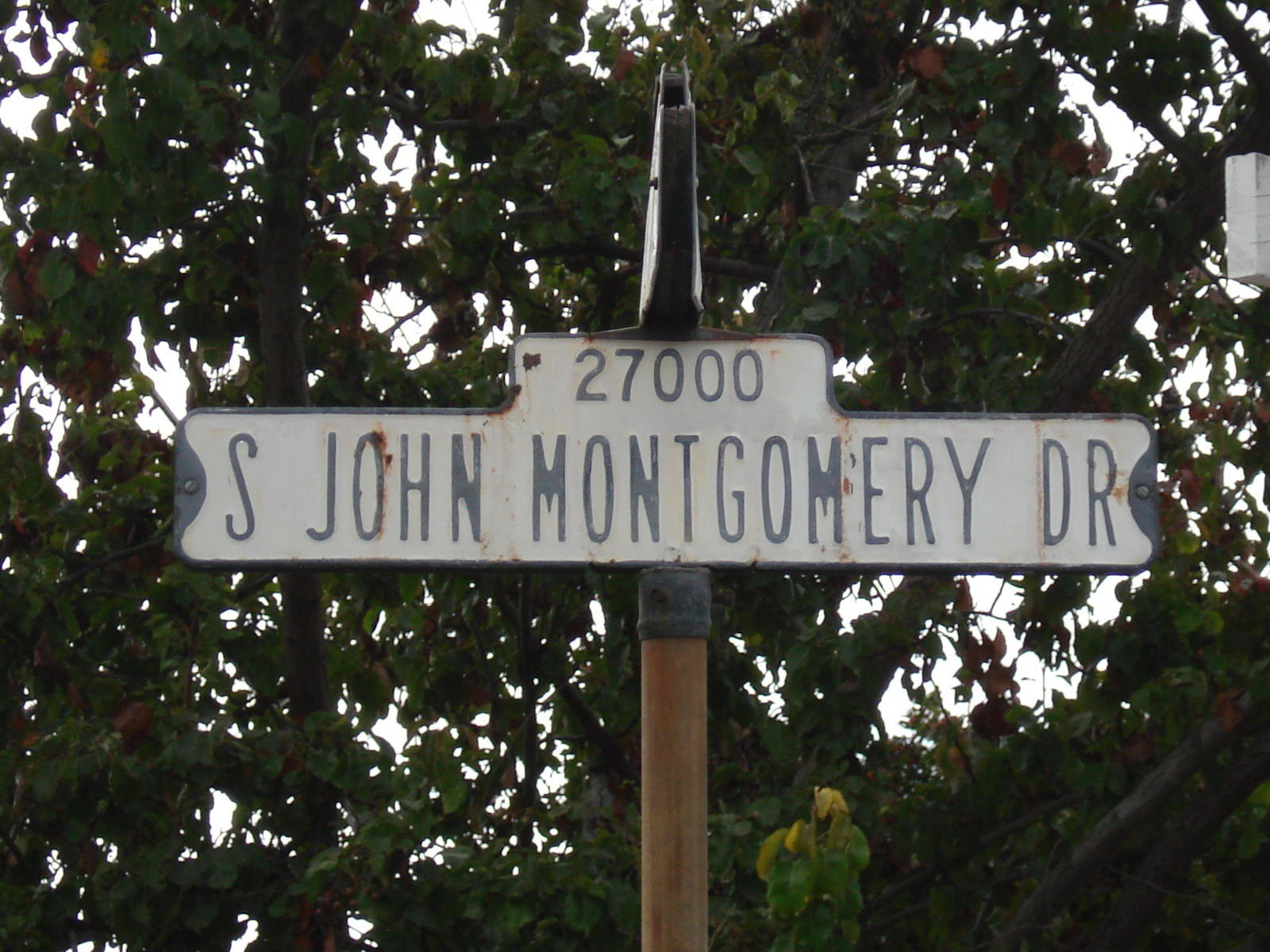The outdoor color photograph captures a weathered street sign mounted on a brown, cylindrical wooden pole with a darker, likely metallic cap on top. The pole shows signs of rust. The street sign consists of two sections: the smaller upper section reads "27000," while the elongated lower section displays "S John Montgomery Dr" in vertically stretched, slightly disproportionate blue-grey lettering, against an off-white background that is peeling and marked by rust in various shades of brown. Notably, in the top left corner of the sign, the peeling has exposed black underneath. Behind the sign, dense green foliage interspersed with reddish-brown and yellowish-green leaves is visible, along with patches of the sky showing through the gaps. Another sign points away from the viewer, hinting at the sign being positioned at an intersection.